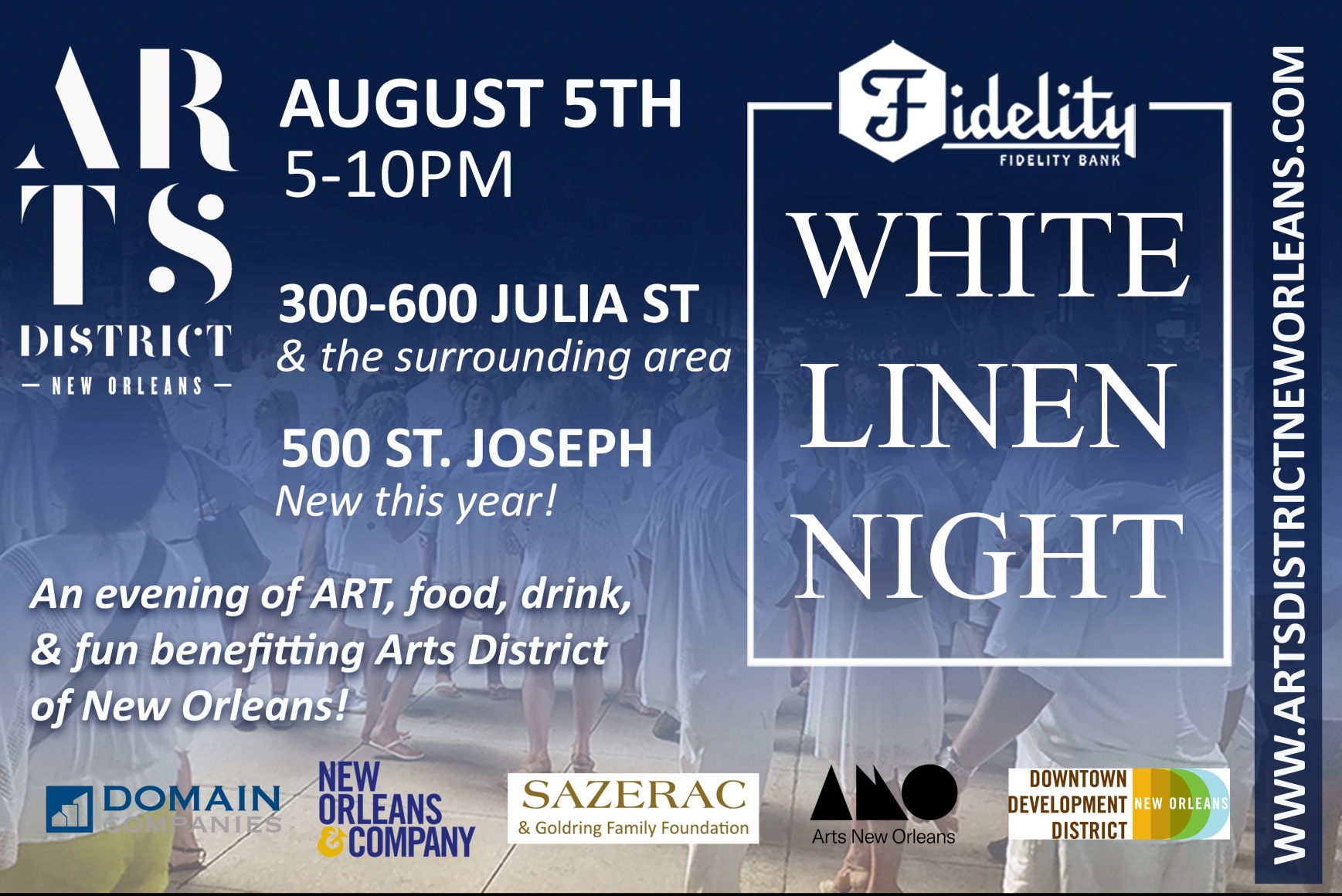The advertisement promotes "White Linen Night," an event benefiting the Arts District of New Orleans. It takes place on August 5th from 5 to 10 pm, spanning 300-600 Julia Street and the surrounding area, with a new location added at 500 St. Joseph. The event features an evening of art, food, drink, and fun. Prominent sponsors include Fidelity Bank, Domain Companies, New Orleans & Company, Sazerac, Gold Ring Family Foundation, Arts New Orleans, and Downtown Development District of New Orleans. The advertisement prominently displays the event details in white text over a blue-tinted, blurred background image of people dressed in white outfits, symbolizing the evening's theme. The website www.artsdistrictneworleans.com is displayed vertically on the right side.